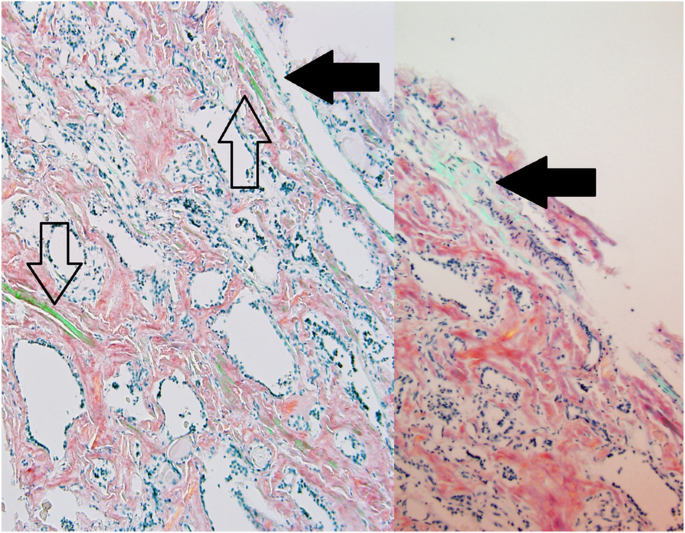This image appears to depict a magnified close-up, potentially of cellular structures, showcasing an array of vibrant, swirling colors. The scene is divided into two asymmetrical sections, with the left side slightly larger than the right. Both sections display a blend of white, blue, pink, and red hues, with various shapes including round, oblong, and squiggly forms.

In the left section, there's a prominent solid black arrow pointing to the left towards a greenish area resembling a vein within the cell. Nearby, another upward-facing arrow has a black border but is transparent in the center, directing attention to a red portion of the slide. Lower on this side, another hollow arrow with a black outline points downwards towards an area with light red, white, and blue swirls, highlighting a long green line.

The right section mirrors the left's swirly and vibrant color scheme, but with a more vivid display. It contains a single solid black arrow pointing left towards a light blue region in the image, echoing the intricate and colorful design observed throughout the composition.